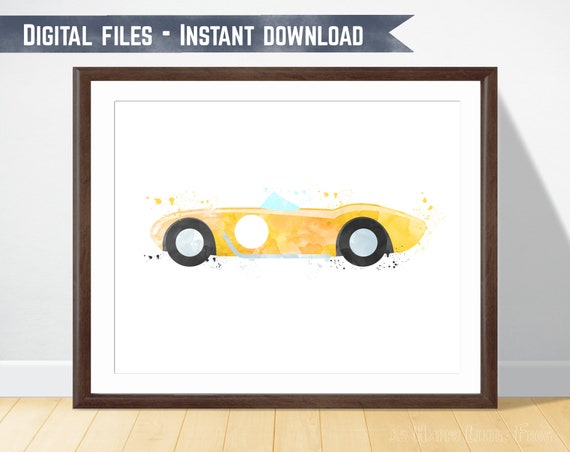The square image features a framed depiction of a yellow sports car, bordered by a dark brown wooden frame with a white backing. The car is presented from a side view, with its front end pointing to the left. The vehicle is a convertible, featuring a bluish-white tinted window. The picture sits upright, leaning against a stark white wall on light wooden flooring, which is partially visible at the bottom of the frame. A text overlay in the upper left-hand corner reads "DIGITAL FILES - INSTANT DOWNLOAD" in all-capital white lettering. The car image itself is somewhat stylized, with yellow speckles that resemble bubbles. Additionally, the black tires and silver rims are noticeable, along with a faint reflection on the side of the frame. The inlay of the frame helps to hold the picture in place, giving the entire presentation a clean and modern aesthetic.